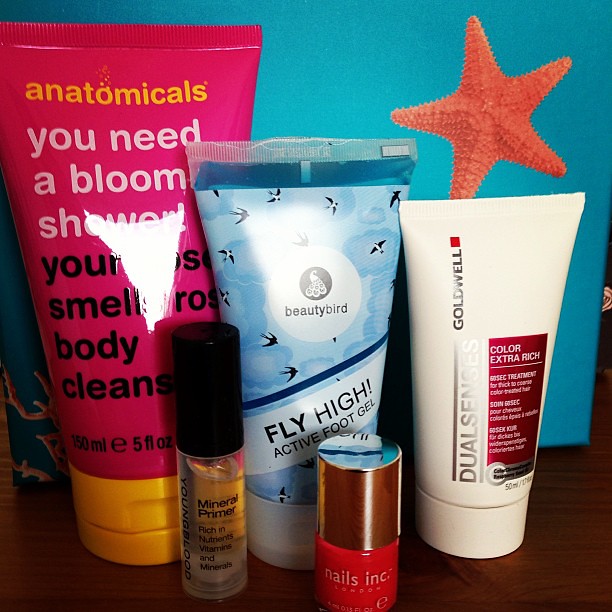Displayed is a colorful and vibrant collection of five beauty products, carefully arranged against a sea-themed background featuring a red starfish and sea plants, all set on a wooden surface. From left to right, we see a pink tube labeled "Anatomicals You Need a Bloom Shower Smelly Rose Body Cleanser." Next is a blue tube branded "Fly High Active Foot Gel." A white tube marked "Goldwell Dual Senses Extra Color Extra Rich" suggests a hair conditioner. In front, there's a bottle of "Nails Inc" red nail polish with a silver cap, and a clear bottle labeled "Mineral Primer." The background's light blue color enhances the array of products, making each item's vibrant hues of yellow, white, pink, blue, red, and brown pop against the serene aquatic setting. The display has a feel of either a subscription box or a well-organized dresser or bathroom.